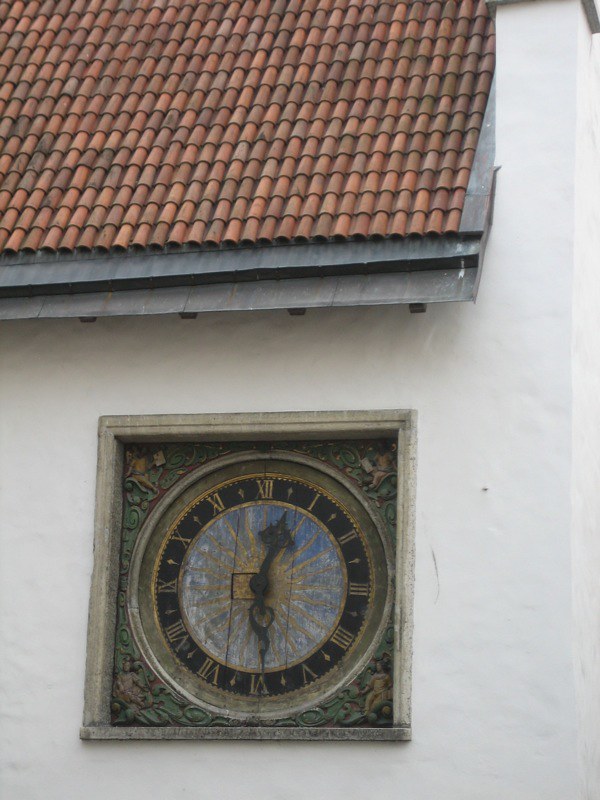The image showcases a striking, light-colored stone building, nearly white in appearance. The roofing, partially visible at the top of the image, features reddish-brown, bamboo-shaped tiles held securely by a surrounding framework, possibly made of another material. Dominating the center of the structure is a large, ornate clock. The clock is encased within a square stone border characterized by a mix of gray, green, and lighter shades. The round clock itself is composed of gray, black, and gold elements, with a striking blue center adorned by a gold sun motif. The clock's design is further enhanced by large, decorative black arms indicating the hour and minute, and a black outer ring embellished with gold Roman numerals.